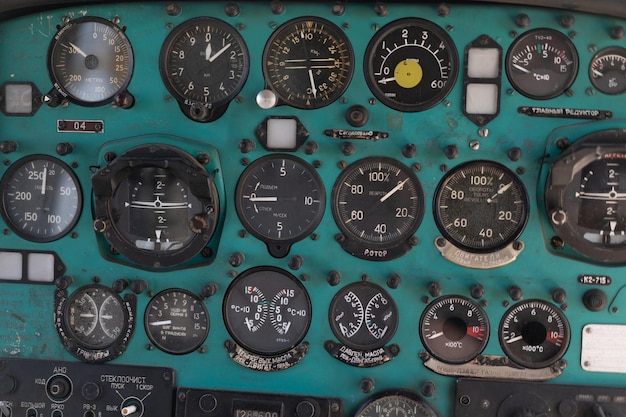The image depicts a highly detailed and photorealistic representation of an instrument panel, likely from an old-fashioned two-seater plane or possibly a boat. The panel is arranged in multiple rows and columns and features a total of about 17 to 18 circular gauges of various readings, primarily pressure measurements. The backdrop is an attractive light aqua blue, creating a stark contrast with the gauges. 

Starting from the top left, there are four evenly-sized black gauges with white numbers. Beside the fourth gauge, a black vertical rectangle contains two white squares. Moving right, there is another gauge with numbers and a white arrow, followed by a smaller black gauge. Across the middle, a black gauge with white numbers and a white arrow stands prominently. Adjacent to this, another black gauge features a white line flanked by the number two above and below it. Next to it, three more black gauges with white numbers are positioned, with the last one in the center also displaying a similar configuration with the number two above and below a white line.

The bottom row consists of six black gauges, all featuring various numbers and white dashes. Among the predominantly black and white gauges, one notable exception includes an orange circle, and a pair of gauges designed to indicate critical measures when in the 'red' zone. The gauges are meticulously aligned on a baseboard which appears greenish in hue. The detailed arrangement and vivid colors contribute to a clear and organized display, essential for precise monitoring in transport modes, specifically aviation.